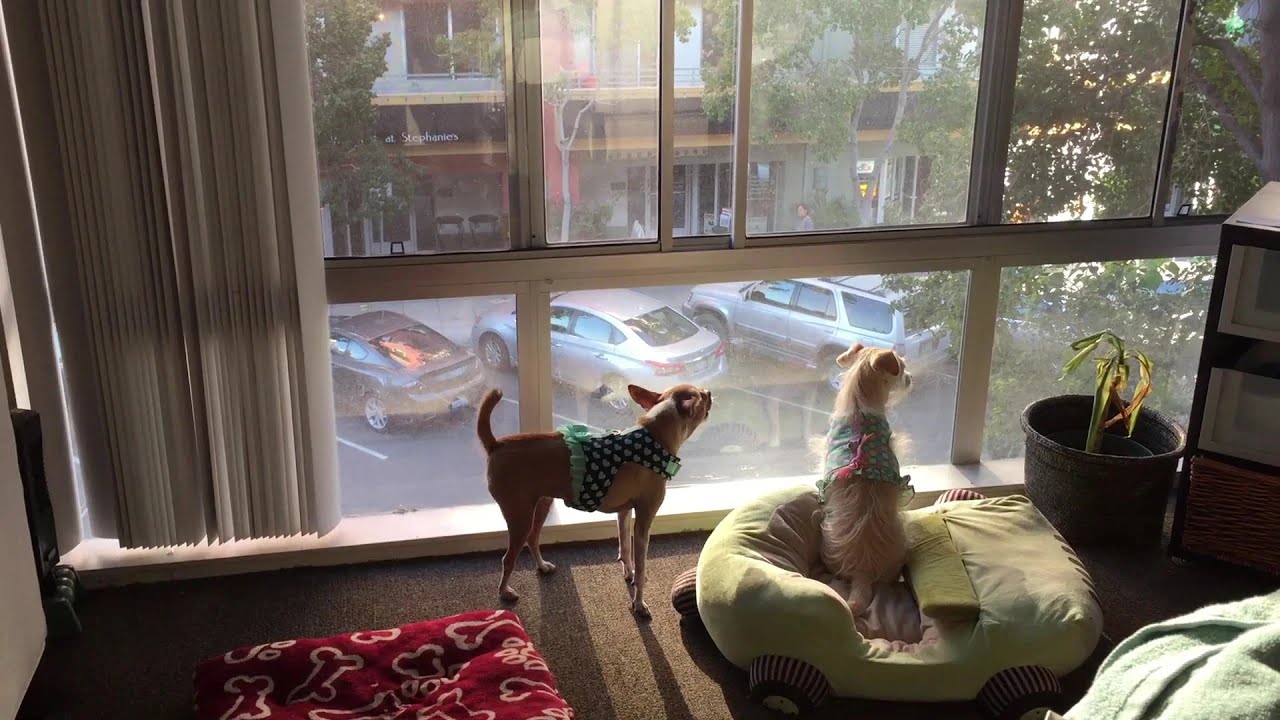In a sunlit, upper-level apartment with large windows and vertical blinds drawn back, two small dogs gaze intently outside. The larger dog, a beige chihuahua with long legs and pointy ears, stands tall, clad in a green and black sweater with ruffles. Just to his right, a lighter beige dog with floppy ears sits comfortably in a plush toy car bed, light green in color, and wears a colorful, pink and green patterned sweater. The window overlooks a parking lot with four visible cars—two silver, one dark gray, and another—parked diagonally below. Across the street lies an adjacent building and some trees. On the right side of the dogs, a large black pot holds a half-dead plant, while on the left, a red dog bed featuring a white and red bone pattern provides additional cozy space. A green towel rests on the bottom right corner of the scene, adding a homely touch to the arrangement.